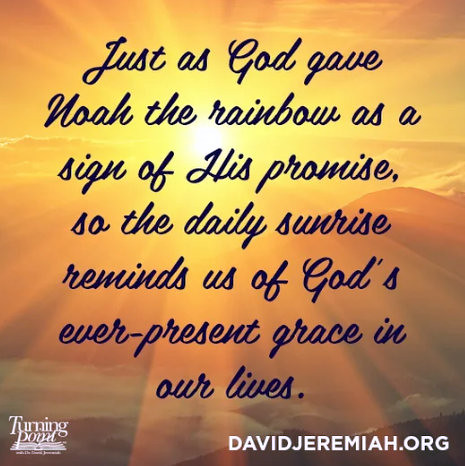This social media-ready inspirational quote graphic features a serene aerial view of mountaintops at sunrise. The center boasts a radiant sunburst with exaggerated bright yellow rays streaming in all directions, which gradually transition to orange, enhancing the depth of the scene. Muted yellow tones dominate the background, allowing black scripty text to stand out with the quote: "Just as God gave Noah the rainbow as a sign of his promise, so the daily sunrise reminds us of God's ever-present grace in our lives." In the lower-left corner, a white Turning Point logo, resembling an open book, adds a subtle touch, while the lower right corner features the URL davidjeremiah.org in white capital letters.